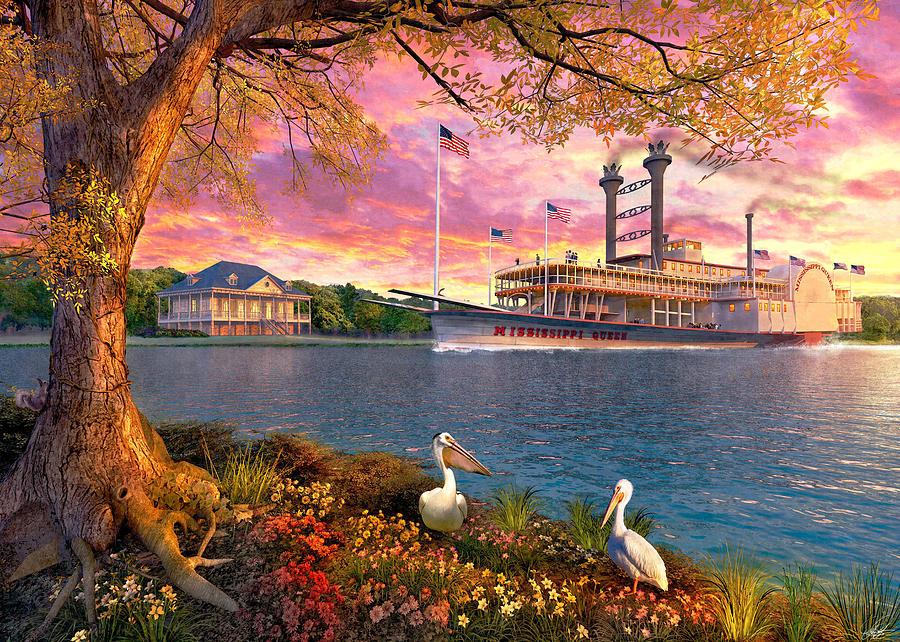In this detailed and vivid painting, we see two pelicans standing on a lush patch of grass in the foreground, directly facing each other amidst an array of colorful, small flowers. The scene is set under a large tree with green leaves that overhangs towards the top of the image, extending a bit above a serene body of water. On the left side of the tree, a squirrel is climbing, adding to the lively atmosphere. 

In the background, on the left side of the riverbank, there is a house, likely a large home, possibly even a plantation, with an American flag flying nearby. The right side of the river features the massive steamboat named Mississippi Queen, a white ship with red text at its base. The steamboat is adorned with numerous American flags, indicating its grandeur and capacity to accommodate many passengers for extended travels. 

The sky above this picturesque scene showcases a beautiful sunset with predominant shades of pink and purple, interspersed with hints of blue and yellow, enhancing the overall tranquil and enchanting quality of the painting.